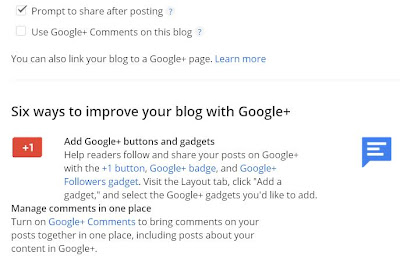In the provided image, we observe a user navigating a blog's settings interface, specifically managing functionalities related to Google Plus integration. At the top of the interface, there's an unchecked option labeled "Prompt to share after posting," which the user has selected. Directly below, another option "Use Google Plus comments on this blog" remains unchecked, indicating the user's disinterest in enabling Google Plus comments.

The page's heading reads "Six Ways to Improve Your Blog with Google Plus," followed by a list of suggested steps. Only two steps are visible in the image:

1. **Add Google Plus buttons and gadgets**: This section contains a small red box featuring the Google Plus logo and the number "+1," alongside a blue quote bubble icon, visually similar to Twitter's design. It suggests utilizing these gadgets to help readers follow and share posts on Google Plus. The recommendation continues with instructions to visit the "Layout" tab, add a gadget, and select the desired Google Plus gadgets.

2. **Manage comments in one place**: Advises enabling Google Plus comments to consolidate all comments, including those from Google Plus posts about the blog content, in a single location. The user has evidently chosen not to enable this feature, as mentioned earlier.

The image illustrates that while the user has interacted with some settings, they have opted not to implement certain Google Plus features, possibly indicating a preference or dissatisfaction with them.